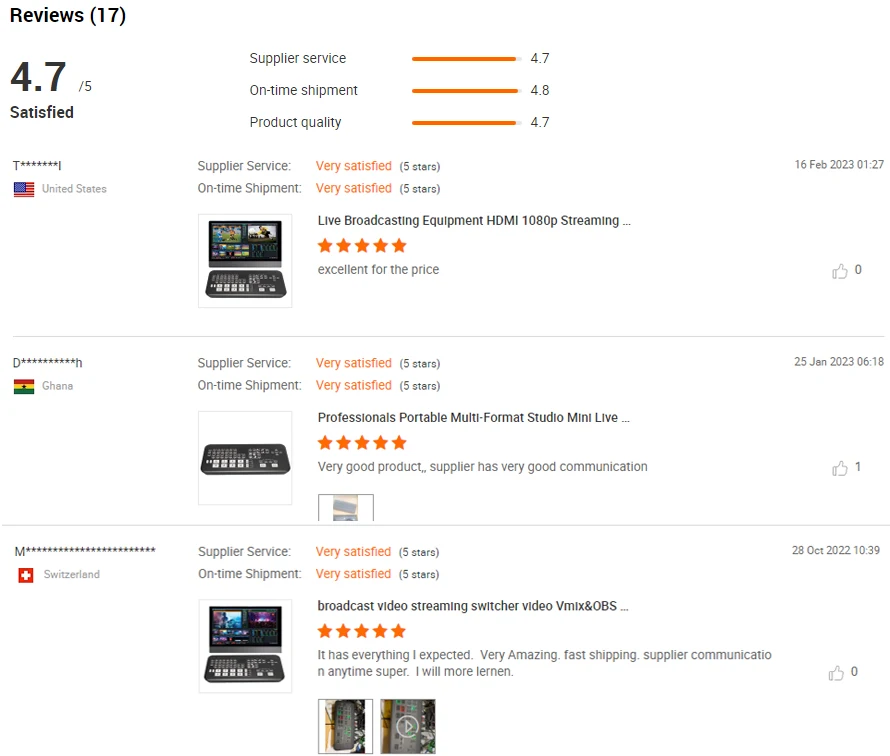A tall, square screenshot appears to show a series of laptop reviews commonly found on an e-commerce platform like Amazon, despite the absence of an Amazon logo. In the upper left corner, it reads "Reviews" in black letters, followed by "(17)" and "4.7/5". Below that, there's an assessment of "Supplier Service" represented by a long orange bar with a bit of gray to the right, rated at 4.7. Directly below, "On-time Shipment" is rated at 4.8, and "Product Quality" at 4.7, both illustrated with similar orange and faint gray bars.

Further down, the image presents three distinct reviews that seem to pertain to various laptops or related devices. The first review, written by an individual from the United States (identified briefly with the initials T*I), rates the product highly. It includes an American flag icon and comments on the supplier service and on-time shipment, each marked as "very satisfied" with five stars. The laptop reviewed is noted as "Live Broadcasting Equipment, HDMI 1080p streaming," with a full five-star rating and the comment "excellent for the price." The review's date is 16 Feb 2023, at 01:27, accompanied by a thumbs-up icon with zero likes.

The second review comes from Ghana (initials D****h), echoing the same satisfaction level. The product here is described as "Professionals Portable Multi-Format Studio Mini Live..." with an overall five-star rating and labeled as a "very good product". The review praises the supplier's communication and notes the date as 25 Jan 2023, at 06:18, and features a thumbs-up with one like.

The final review is by a reviewer from Switzerland (initial M******), again rating the supplier service and on-time shipment at full satisfaction. The product here is designated as "Broadcast Video Streaming Switcher Video, vMix and OBS..." with complete five stars. The comment highlights the product met expectations, with "very amazing, fast shipping, supplier communication," and features "I will learn" cut off at the end. Additional images of the product, likely a laptop or keyboard, are shown, with one having a white play button indicating a video. This review is dated 28 Oct 2022, at 10:39, accompanied by a thumbs-up icon with zero likes.

Overall, the image appears to provide a comprehensive overview of various highly-rated products, likely laptops or related broadcasting equipment, with detailed user reviews and ratings on an online shopping platform.